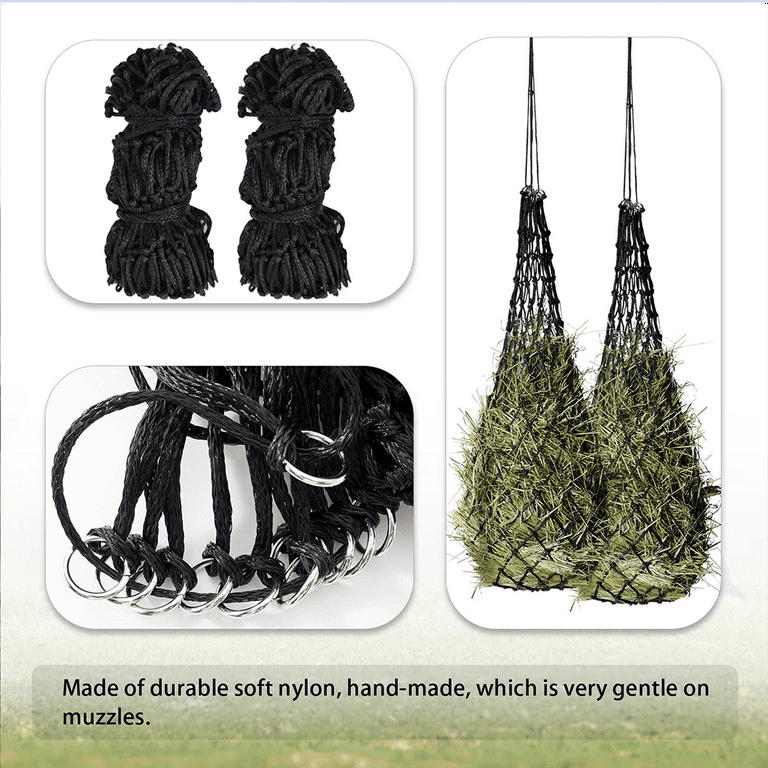This is a real-life photograph comprising three images, potentially from an advertisement or catalog. The top image depicts two black, coiled hanging baskets, possibly made using a neon-like loop for the hanging mechanism. The middle image provides an up-close view of the silver rings and the durable, soft nylon material of the baskets. The bottom image shows the baskets in use, each holding hay or grass and displayed hanging, offering a full view of their function. The accompanying text indicates that the baskets are "made of durable soft nylon, handmade, which is very gentle on muzzles." This suggests that the baskets are designed as a feeding device for horses or cows, providing a gentle and practical means for animals to feed.